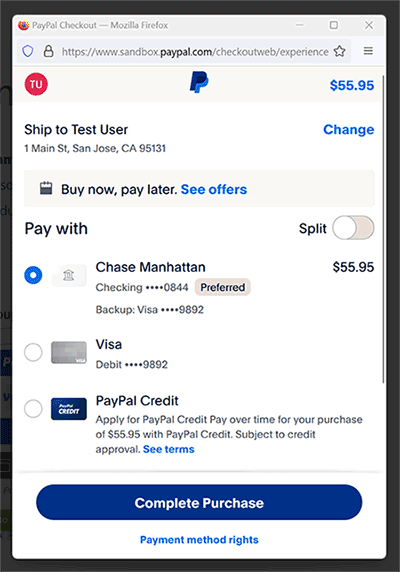In the background, the borders are gray. The top left corner features a variety of elements including a PayPal checkout interface within the Mozilla Firefox browser. There is a blue shield icon and a lock symbol beside the URL, which reads "https://sandbox.paypal.com/checkout/web/experience". Nearby, there is a star icon and a hamburger menu. 

A prominent red circle is also visible. The interface displays the PayPal logo featuring a dark blue 'P' interlaced with a light blue 'P'. The amount of $55.95 is shown in blue text. The address listed is "Shift to test user, 1 Main Street, San Jose, California, 95131" with an option to "Change" it in blue text. There is a calendar indicating a "Buy Now, Pay Later" option with blue text prompting to "See Offers". 

To the right, the payment method section displays a blue check mark next to "Chase Manhattan Checking ....0844, preferred", followed by a "backup Visa ....9892" option and a "Visa Debit ....9892, $55.95" option. PayPal Credit is also mentioned but not selected, with blue text stating "PayPal Credit: Apply for PayPal Credit, pay overtime for your purchase of $55.95 with PayPal Credit". The screen concludes with a "Complete Purchase" button.